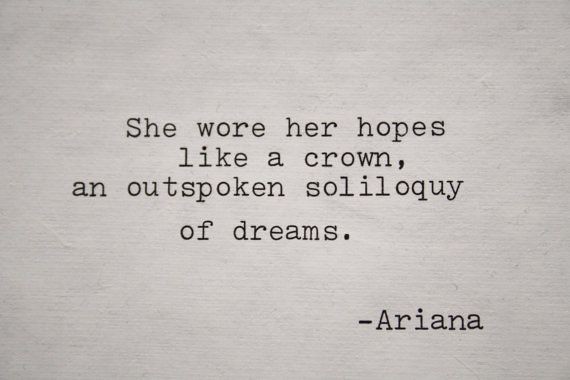A visually compelling image features a literary quote presented in typewriter font, centrally positioned on a slightly wrinkled, gray piece of paper. The prominent quote reads, "She wore her hopes like a crown, an outspoken soliloquy of dreams." The author's name, Ariana, is discreetly placed in the lower right corner, marked in a smaller font size. The subtle horizontal wrinkles give the paper a textured, organic feel, adding depth and character to the minimalistic composition.